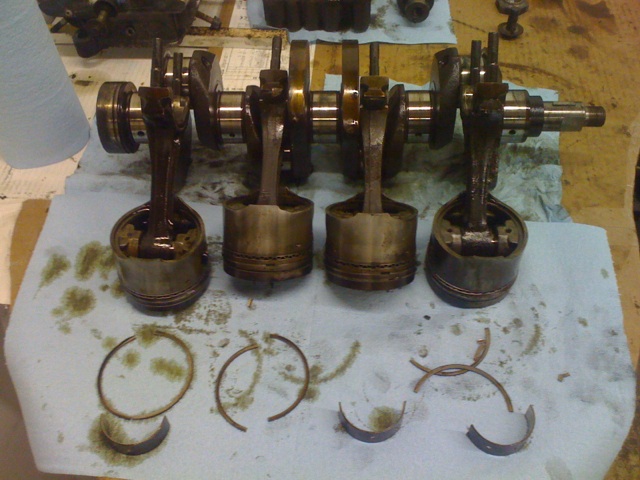The photograph depicts a set of old, oil-covered engine pistons, each with a brownish appearance, meticulously arranged on a white piece of cardboard that is marred by multiple oil stains. These piston components, typically integral to an engine, are presently detached and are connected to a heavy, long metal rod, signifying their usual role in the rotational mechanism of the engine. In the forefront, there are several warped and broken gaskets that were once circular metal rings, but are now mostly split in half, adding to the visual of mechanical wear and age. Additional engine parts are scattered in the background, placed on either more pieces of cardboard or blue paper towels, contributing to the industrial, workshop setting of the image.